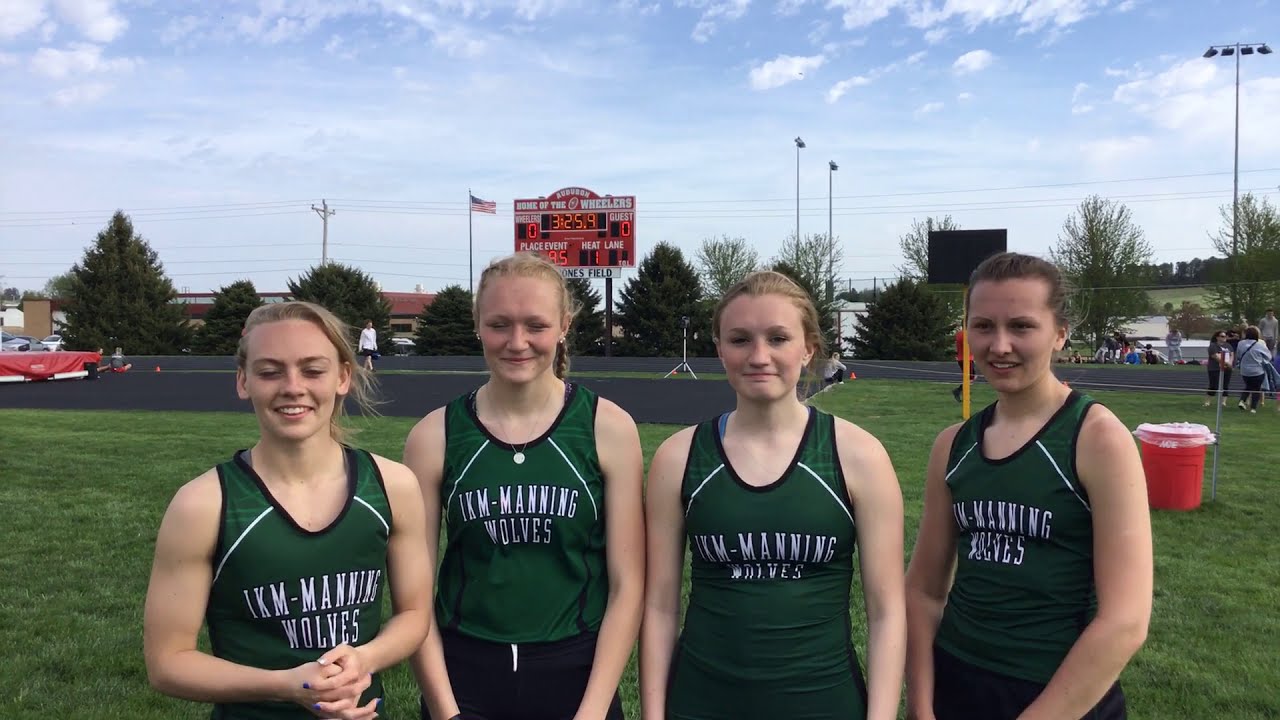In this outdoor image, we see four young female athletes, likely runners from a track and field team, posing for a photo on a sports field. They are dressed in matching green sleeveless jerseys with white text that reads "IKM-Manning Wolves," and they are also wearing black shorts. All the girls have their hair pulled back in ponytails and are smiling for the camera—well, most of them are. They stand on a grassy infield area that appears to be part of a track meet setup, evident by the high jump mat and scattered ropes around them. 

Behind the athletes, there is a scoreboard that reads "Home of the Wheelers" with a score of 0-0 and "Heat One" displayed, indicating the ongoing event. The timer shows three minutes and two seconds remaining. Further back, we notice an orange garbage bucket, some light poles, a flag, and a parking lot, all framed by a line of trees. The sky stretches out above with a few clouds dotting the blue expanse. The field and surroundings give a lively sense of a bright, clear day, capturing the essence of a competitive sports environment.